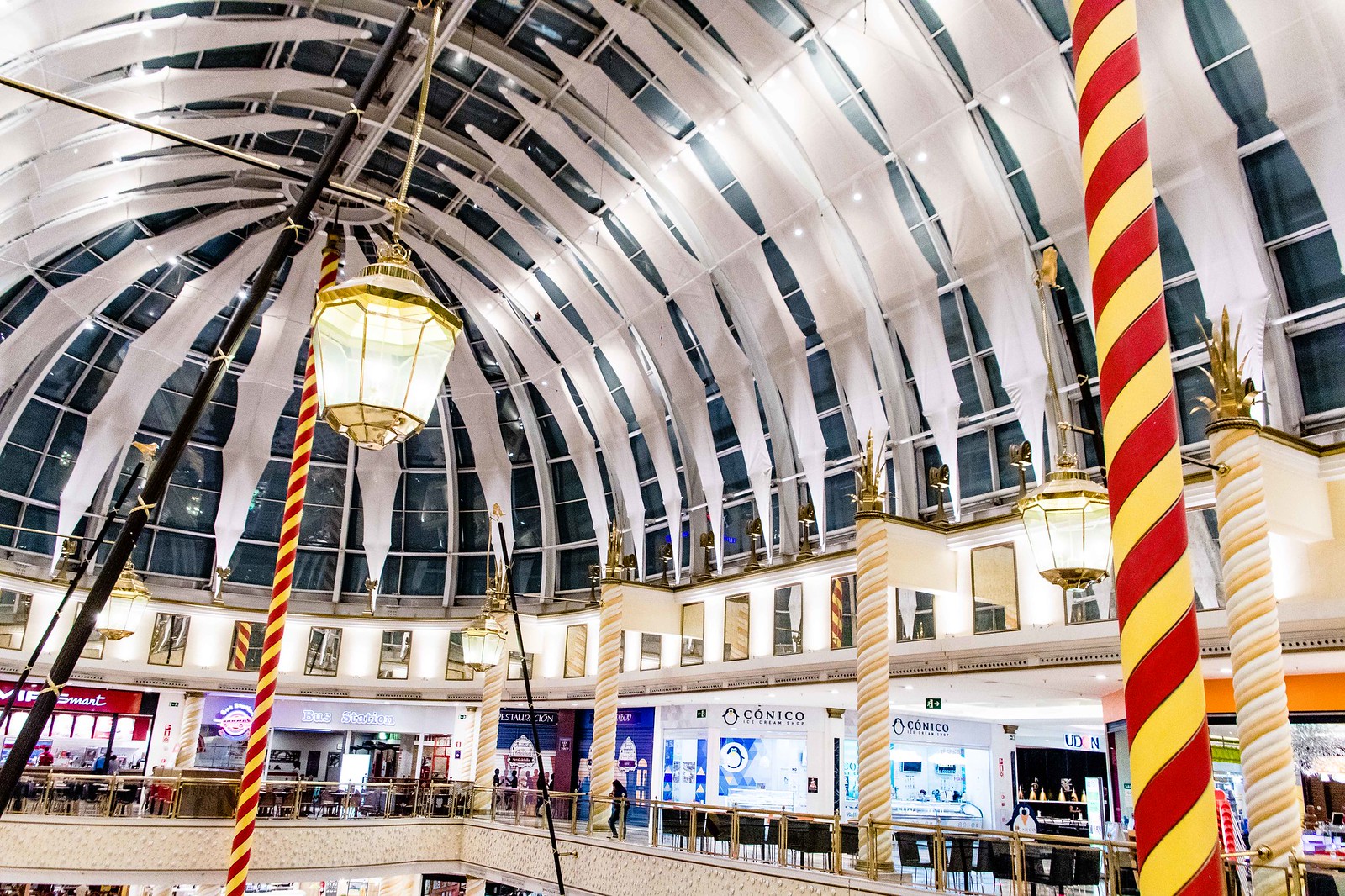The photograph captures an opulent, expansive shopping mall viewed from an upper level, focusing on a grand domed ceiling made of glass. The dome structure is lined with elegant white, rib-like arches that give it a rib cage appearance. Hanging centrally from the ceiling is a distinctive light fixture that resembles a pendulum. Below the dome, columns striped in red and yellow stand out, reminiscent of festive candy canes, suggesting a possible Christmastime setting. The space is adorned with gold and white decor, enhancing its luxurious feel. Numerous storefronts line the upper floor, with some recognizable ones such as "Conoco." The scene is devoid of people, spotlighting the architectural beauty and opulence of the mall, which includes seating areas that resemble small restaurants and a few jewelry stores on the right side.